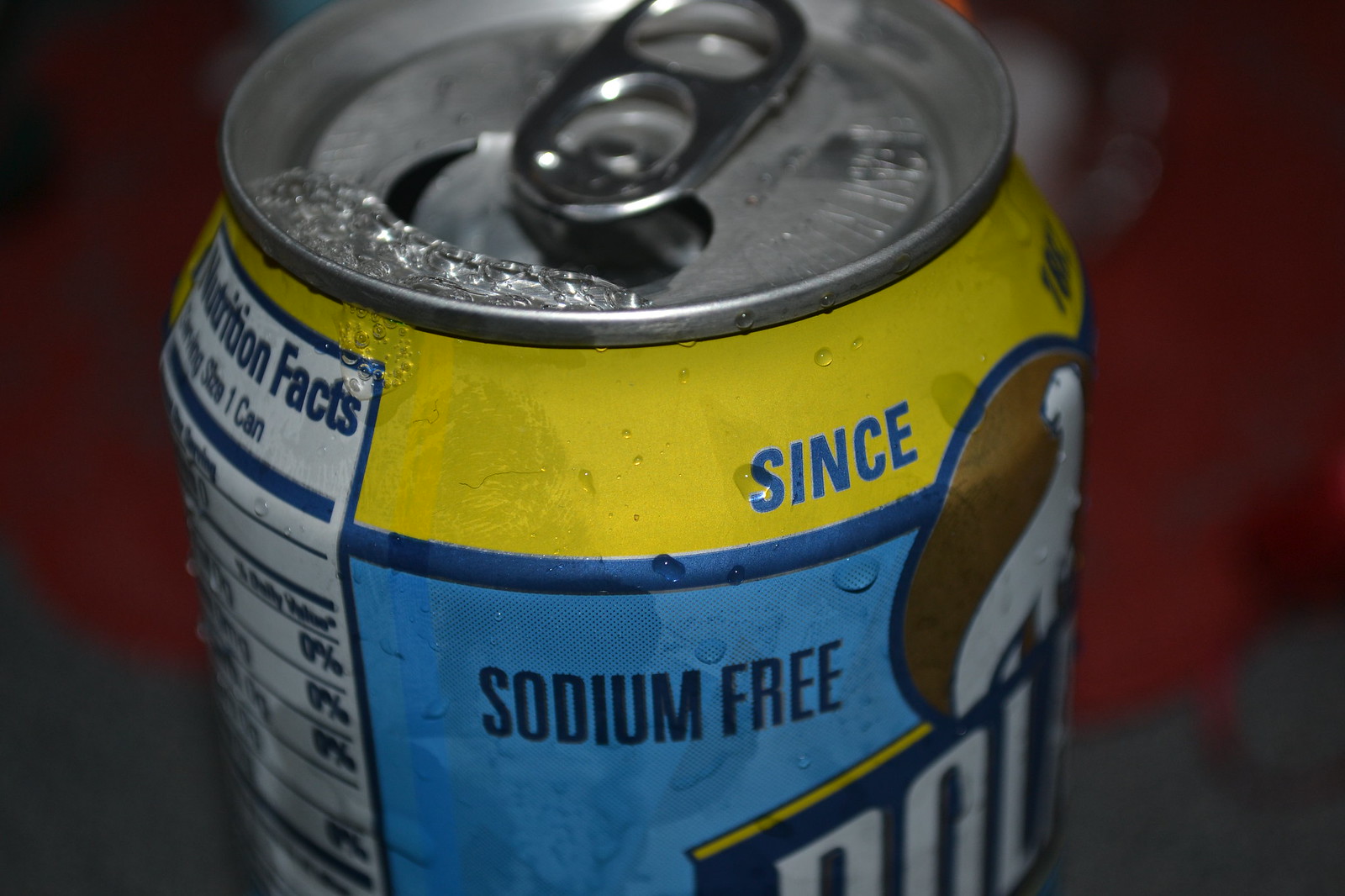The image displays a close-up of the top portion of an open can, prominently featuring an aluminum design. The can is primarily blue with a yellow ring encircling the top. On this yellow ring, the partially visible word "since" is written, hinting at an unseen date. Below this, in the blue section of the can, the term "sodium-free" is clearly printed. Near the top opening, some ice remnants and condensation are visible, indicating that the can has recently been chilled and is now sweating slightly. 

Fingerprints can be seen around the can's opening, suggesting it has already been handled and possibly drunk from. Adjacent to the yellow and blue area, there’s a partial view of the nutritional facts table on the left side, mostly showing zeros in the daily values. The can also displays a logo near the base, featuring a polar bear within a brown circle, with additional dark blue text outlined in yellow, likely reading "Polar," though it's not completely visible. The blurred red and grayish background occupies most of the frame, providing a contrasting backdrop to the prominently featured can.